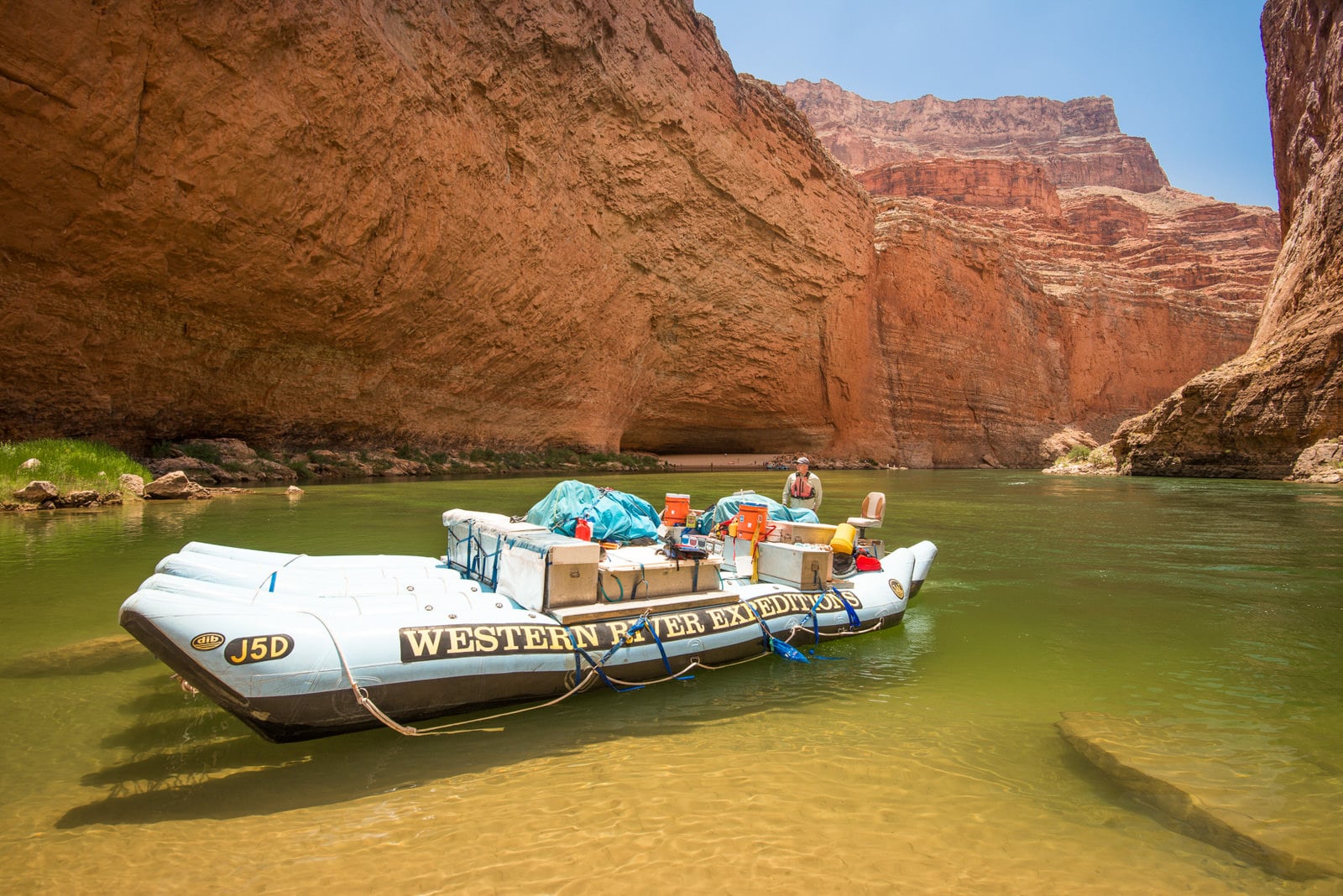This full-color photograph, taken on a bright, sunny day, captures the serene and majestic landscape of the Grand Canyon from the perspective of the Colorado River. The image is horizontally rectangular with no specific border. Dominating the top half of the photo are sheer, dark reddish-brown cliffs of the Grand Canyon that rise steeply, revealing a clear blue sky devoid of clouds in the upper right-hand corner. The lower half showcases the calm, greenish-hued waters of the Colorado River. Centrally featured is a large, white inflatable raft with "Western River Expeditions" emblazoned in yellow, capital letters along the side. The boat is laden with various boxes, trunks, and tarps, suggesting a supply expedition. A guide, clad in a long-sleeved khaki outfit and matching hat, stands at the rear of the raft next to a prominent leather seat, poised as if preparing to bring supplies to shore. The overall scene is framed by the vast and awe-inspiring walls of the canyon, which in the distance transition into mesa-like, flat-topped formations.